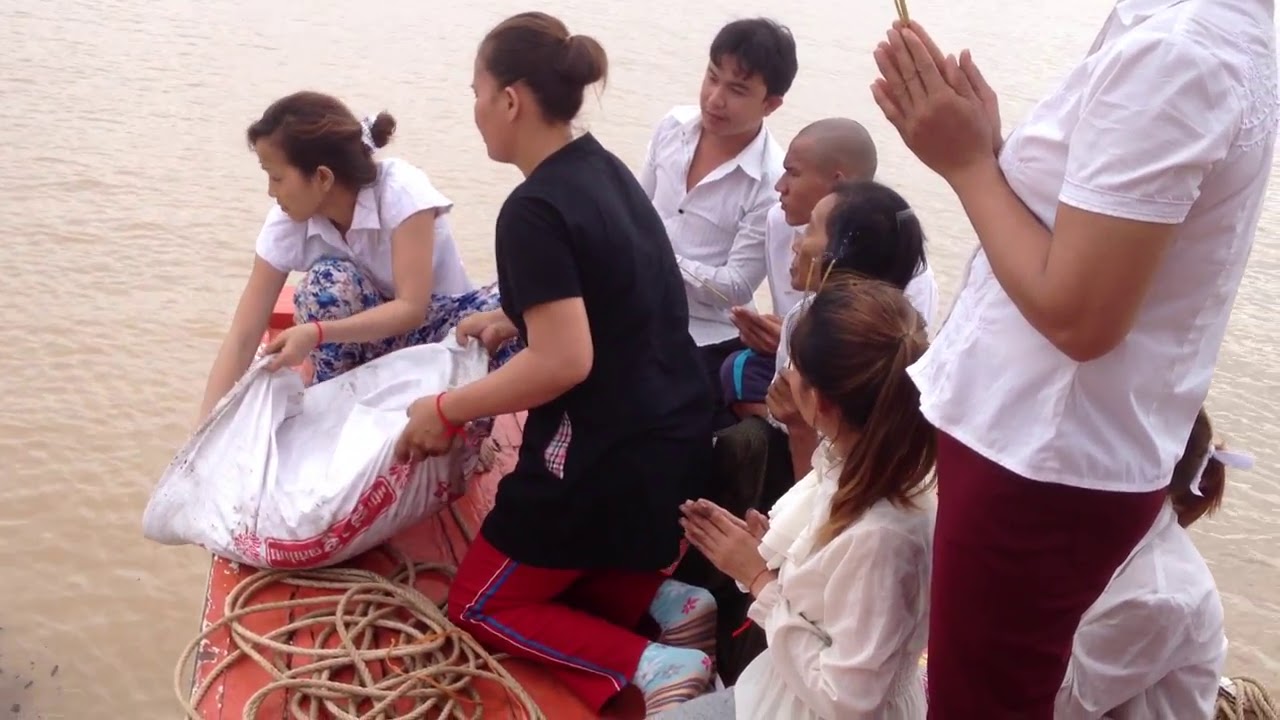The photograph captures a group of eight individuals, predominantly of Asian descent, gathered on a red wooden dock protruding over murky, brownish water that resembles the color of dirty coffee. The group includes both males and females, with most individuals wearing white tops, while one female stands out in all-black attire paired with a red wristband. Another noticeable figure is a woman in a white shirt and crimson red pants, whose upper body is cropped out of the frame. 

The setting is detailed with a light brown rope lying on the dock, which adds a rustic texture to the scene. Among the group, two women are prominently positioned as they tilt a large, white sack towards the water, possibly emptying its contents, although nothing is visibly flowing from the sack. This activity draws the attention of onlookers, with some of the group members sitting or kneeling with hands together, giving the impression of a collective, possibly ritualistic action. The water reflects sunlight, emphasizing its murky quality, while the wooden structure of the dock, although partially obscured by the people, anchors the scene with its vibrant red hue.